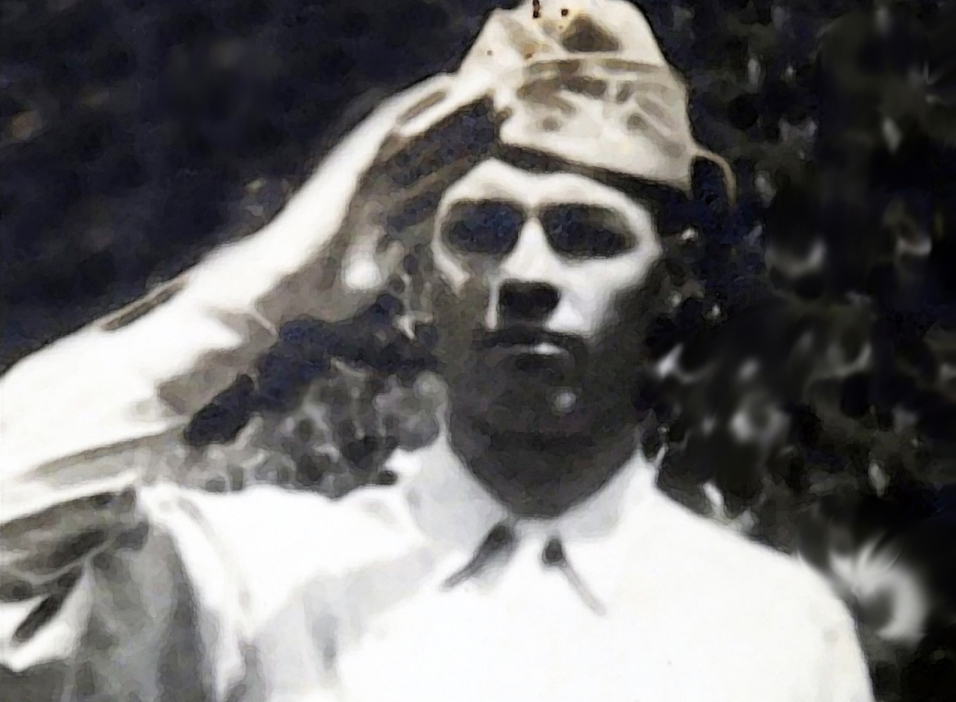This is a very old black and white photograph, potentially from the 1930s, featuring a stern-looking Caucasian soldier saluting with his right hand raised to his forehead. The soldier's expression is serious, with no smile, and his eyes are obscured, adding a mysterious and slightly eerie element to the image. He wears an army-type cap and a buttoned-up white collared shirt, possibly accompanied by a tie. The photograph quality is very poor, with the background appearing as a black void with indistinct gray and white areas, further emphasizing the solitary figure of the soldier. The unclear, wavy backdrop heightens the enigmatic and somber mood of the scene.